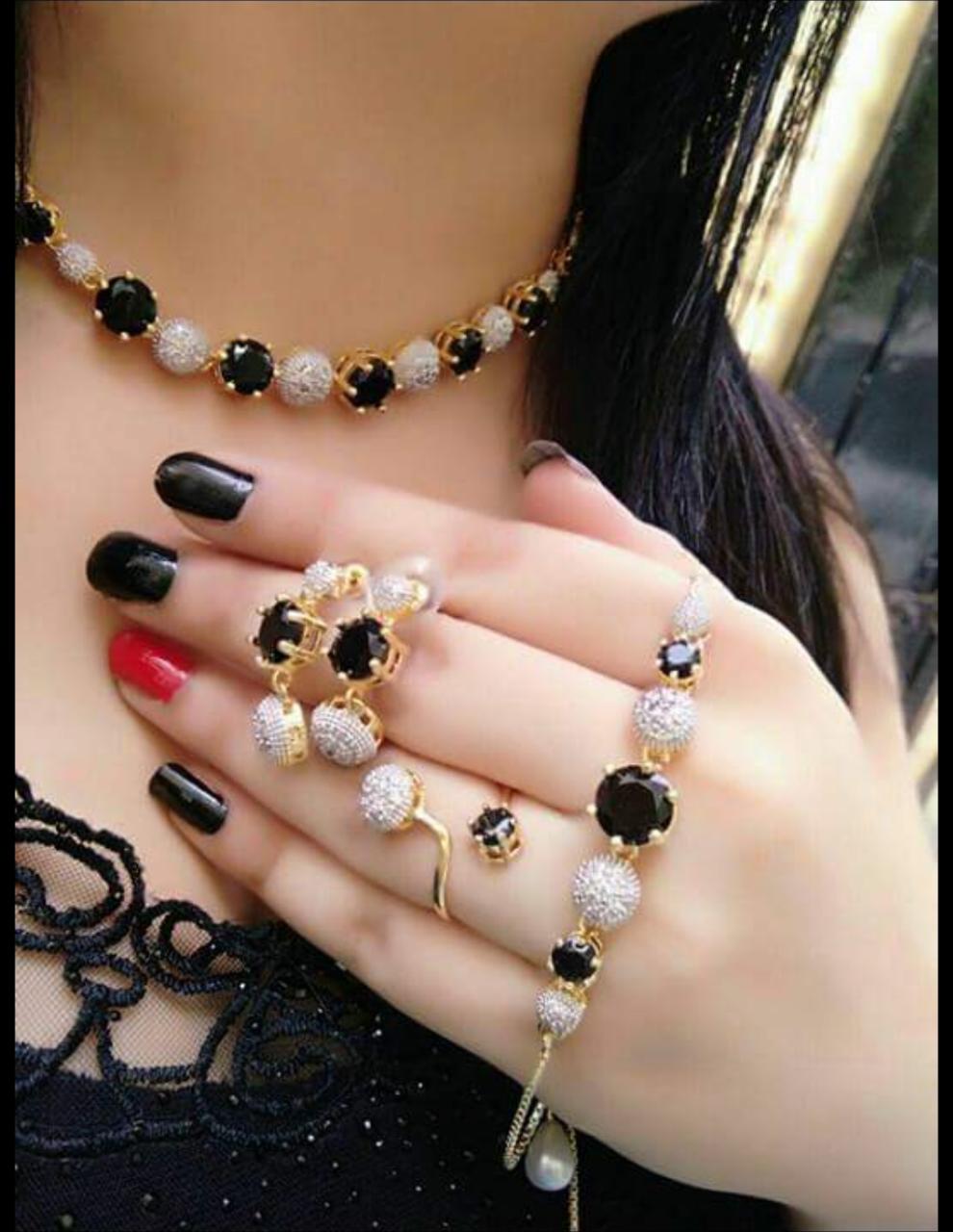This detailed photograph captures a woman with long, straight black hair, against a dark background with hints of a large white chair behind her. Dressed in a black top, her exquisite jewelry stands out remarkably. Around her neck is a striking necklace composed of alternating black gemstones and shiny silver or opal-like beads, all encased in a delicate gold casing. Similarly, elegant pieces of jewelry—mirroring the design of the necklace—adorn her hand and fingers. She wears a matching bracelet around the base of her fingers, and two additional rings showcasing the same pattern of black and silver beads set in gold. Her neatly manicured nails are predominantly painted black, with one middle finger showcasing a bold red polish, resting across her chest and adding a pop of color to the elegant ensemble.